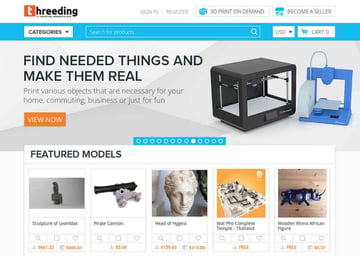The image depicts a screenshot of the website "threeding.com." The website's logo is displayed prominently, featuring a lowercase "t" in white text within an orange square, followed by "hreeding" in black font. There are buttons for signing in and for becoming a seller, alongside a slogan that reads "3D Print on Demand."

At the top of the site, a blue rectangle contains a white drop-down box labeled "Categories," a search bar, and a cart icon. Below this header, the site encourages users to "Find needed things and make them real," signifying its focus on 3D printing.

The main section of the website showcases "Featured Models," including a sculpture of an unknown subject, a "Pirate Cannon," a head statue, a diorama, and a pair of goggles set against a wood background. The overall design of the website, while detailed, presents difficulties in readability due to small font size and intricacy.